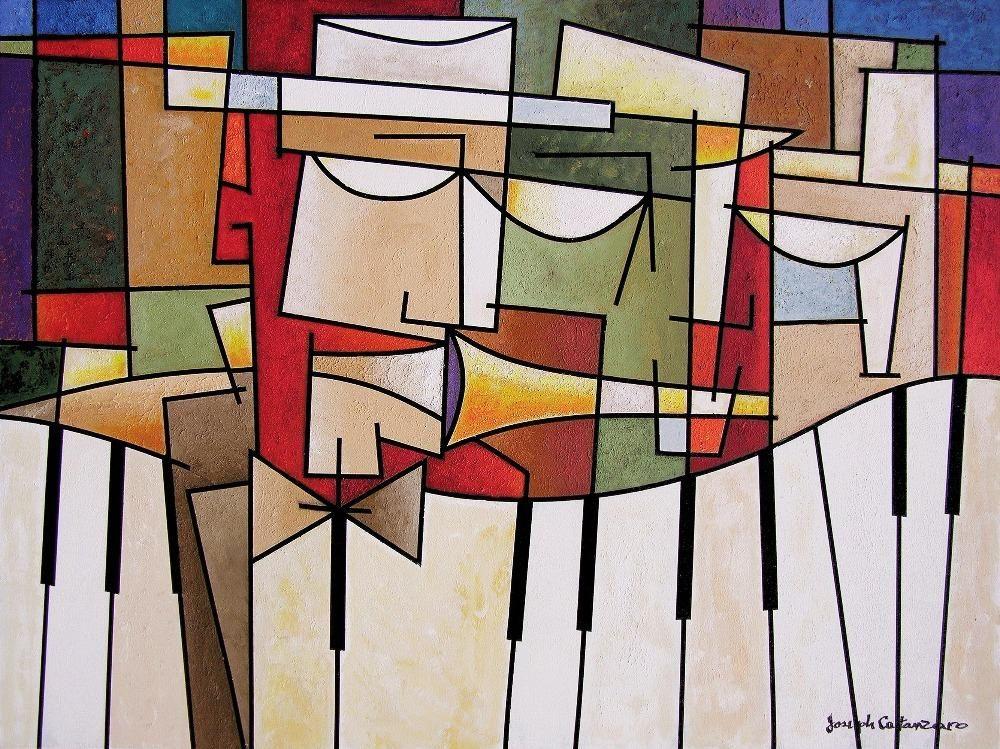This vibrant, expressionist painting by Joseph Cantazzaro features a dynamic and colorful composition. The bottom of the artwork showcases a curved pattern reminiscent of a piano keyboard, with slender black lines morphing into broader shapes, interspersed with yellowish hues. Above this undulating base, a kaleidoscope of geometric shapes—ranging from squares and triangles to oblong rectangles—creates a visual tapestry. These shapes, each uniquely colored in shades of red, orange, green, blue, and more, seem to merge and overlap in an abstract manner. Amidst the chaos, some shapes form facial-like figures. One prominent figure, possibly wearing a cowboy hat, appears to have a red chin and ears, and is positioned next to another face with a green complexion and a hat tilted downwards, seemingly playing a trumpet. The scattering of colors and forms evokes a sense of rhythmic movement and musicality, resonating with the theme suggested by the piano keys at the bottom. The complexity and abstract nature of the painting make it a compelling piece of expressionist art, inviting personal interpretation and engagement.